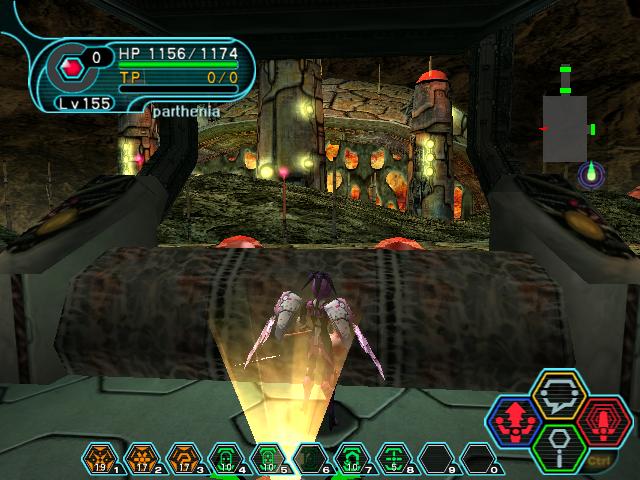This screenshot captures an immersive, dark-themed video game scene centered around a striking character. The character, resembling a dark angel, stands prominently at the bottom-center of the screen. He is adorned with white wings accented with black, resembling spiky hair, and is clad in a black suit with purple highlights. A mysterious yellow light illuminates him from below, casting an eerie glow. He stands on an octagonal platform, with a large round barrier in front of him, surrounded by elements like a pink torch and dirt, suggesting a cave-like environment.

In the top-left corner of the screen is the stats bar displaying "HP 1156/1174" and "TP 0/0." The bar is filled with green, indicating the character's health points. Just below it, in small white letters, it reads "LV 155" and "Parthenia." The bottom of the screen features an action bar comprised of hexagonal icons, each representing different abilities or items. The icons display numbers such as 19, 17, 17, 10, 10, and more, with some slots blank. The bottom-right corner houses a directional pad and additional items like chat and a microphone symbol. The overall scene suggests an intense, fantasy adventure set in a dark world.